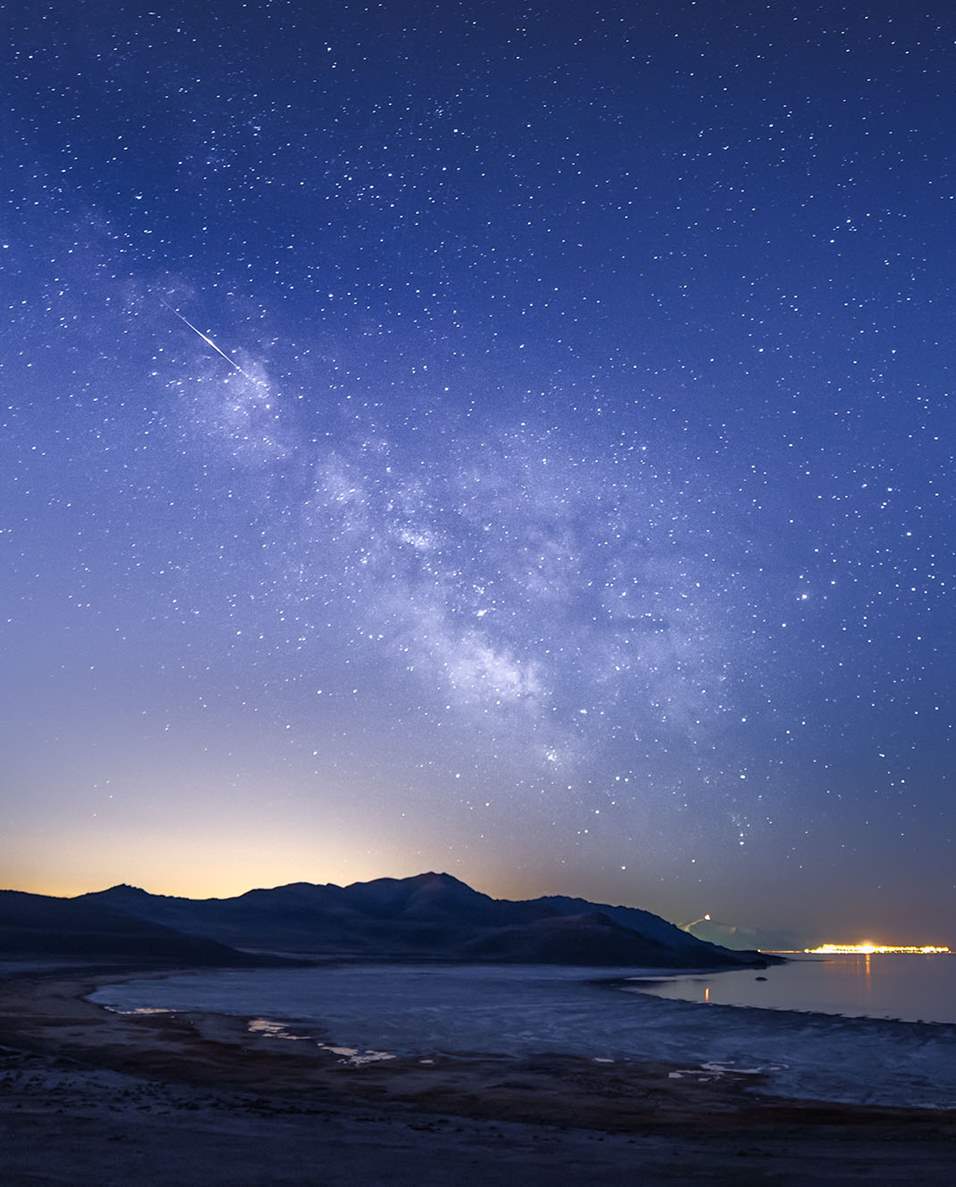This captivating image features a beach adjacent to what appears to be a serene lake, set against a backdrop of majestic hills or mountains. The composition is striking, with the sun setting and casting a warm glow across the scene, indicative of dusk. Yet, intriguingly, the sky remains a vibrant blue, interspersed with an awe-inspiring display of the Milky Way and myriad stars, creating a dreamlike juxtaposition that suggests either a long exposure or a composite of multiple images.

Farther out, the glimmer of bright city lights can be seen, illuminating the distant horizon and adding a touch of civilization to the otherwise natural landscape. The overall effect is a harmonious blend of celestial and terrestrial elements—a beach or bay outlook that somehow captures both the end of day and the profundity of a starlit night. The mix of natural beauty and possibly manipulated imagery leaves one pondering the medium, be it photograph, painting, or digital creation. This enchanting picture masterfully combines the stunning colors of dusk, serene waters, dramatic highlands, and the infinite expanse of the universe, making it an extraordinary visual experience.